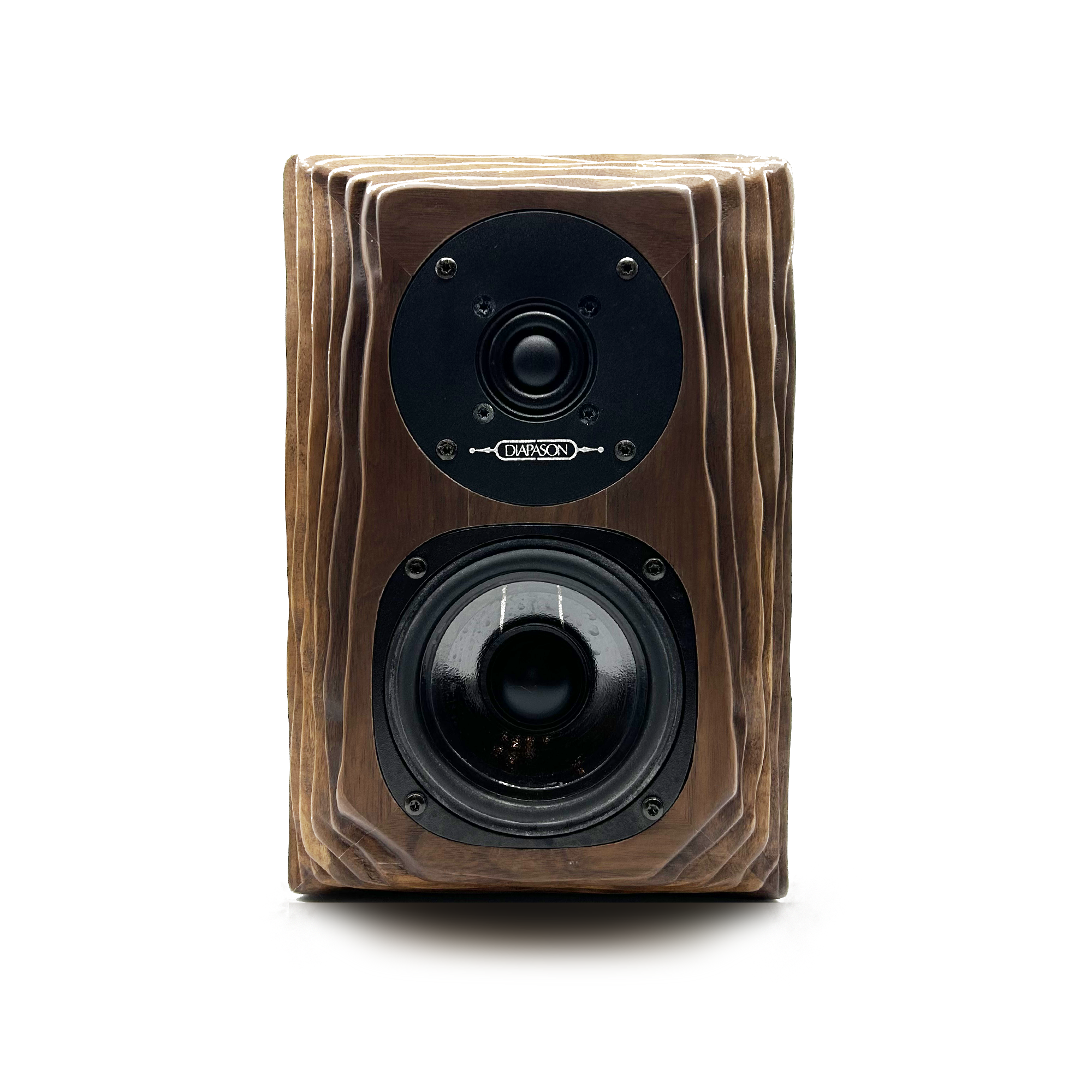The image depicts a vertical, rectangular speaker system made of dark, rich brown wood, resembling a carved tree stump with multiple layered edges that step inward, creating a textured appearance. The speaker is carefully paneled and features two main speaker heads, or subwoofers, stacked vertically in the center. 

At the top half, there is a prominent black circular component, encircled by four screws positioned at each corner—top left, top right, bottom left, and bottom right—encasing what appears to be a rubber button in the middle. This circle also has an inner circle within it. Below this, on the bottom half, there's another similar black circle, with a circular plastic element on top and four screws arranged similarly. The top speaker is labeled "Dypson."

A distinct shadow casts from the bottom of the speaker, enhancing the three-dimensional aspect of the design.